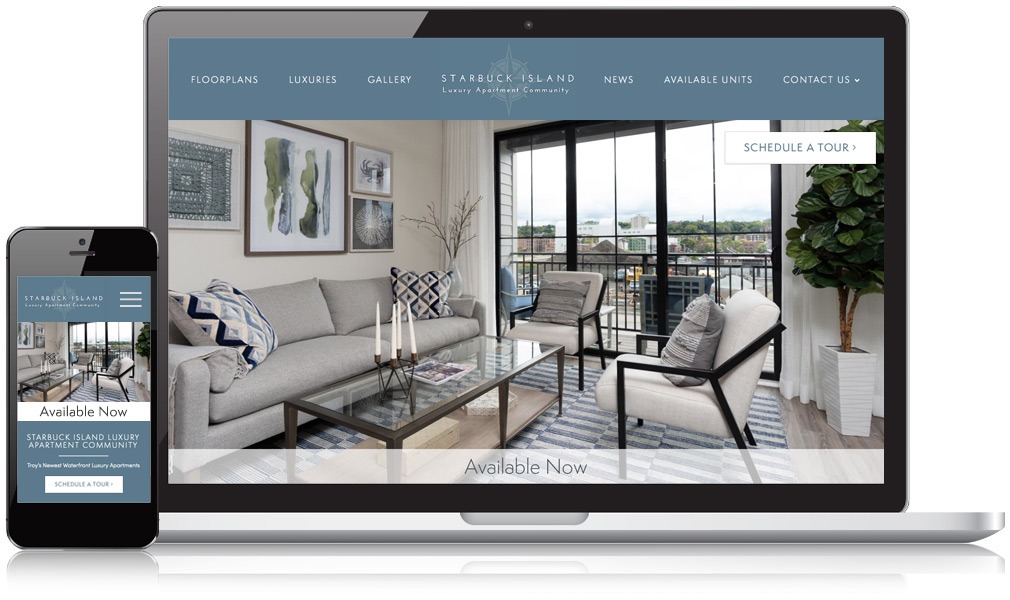On the left side of the image, a mobile phone screen displays the mobile version of a website dedicated to showcasing apartments in the Starbuck Island Luxury Apartment Community. On the right, a larger screen, likely that of a laptop or tablet, exhibits the desktop version of the same website. Both versions feature a consistent blue banner across the top, with white text listing navigational options from left to right: "Floor Plans," "Luxuries," and "Gallery." Centrally positioned within the banner, the text reads "Starbuck Island Luxury Apartment Community" accompanied by a white compass icon. To the right, additional menu options include "News," "Available Units," and "Contact Us," with an arrow indicating a drop-down menu.

Below the navigation banner, an image of a modern living room is prominently displayed. The living room boasts white walls and floor-to-ceiling glass patio doors that lead to a balcony, offering a view of the street and neighboring buildings in the city. The room features a glass top coffee table, a blue and white striped rug atop wood flooring, a gray couch paired with white armchairs, and accent pillows in gray and white. Wall art in elegant frames adorns the walls, adding a touch of sophistication. A large white planter holds a potted plant, possibly artificial, and a side table hosts a vase filled with decorative branches. A clickable box labeled "Schedule a Tour" and a banner at the bottom of the image stating "Available Now" indicate the website's purpose in advertising available units in this upscale apartment community.

This website impeccably highlights the available units and amenities of the Starbuck Island Luxury Apartment Community, providing a seamless browsing experience across mobile and desktop platforms.